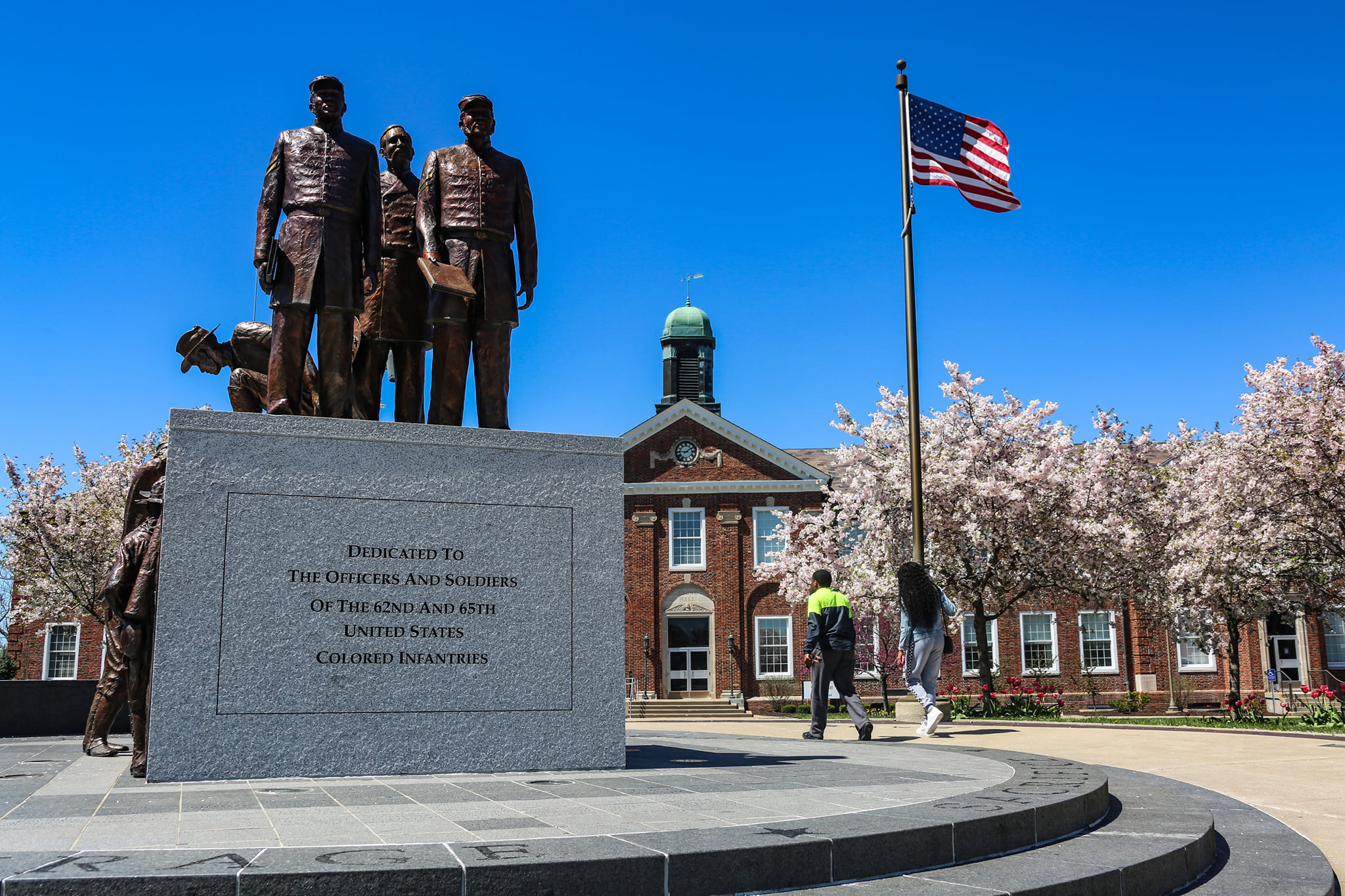In this vibrant photograph, we see a striking statue outside a red brick museum, potentially a Civil War museum, under a clear, blue sky. The scene is dominated by a monument dedicated to the officers and soldiers of the 62nd and 65th United States Colored Infantries, as inscribed in all capital letters on its substantial, gray granite base. The monument, set atop a circular base with granite steps, features four African American men in Civil War-era uniforms. Three of the figures stand erect, each holding a book, while one kneels behind them, appearing to offer assistance.

In the foreground, two visitors, a woman in a blue dress and white sneakers and a man in a fluorescent green jacket, walk toward the museum. This red brick building, with at least two stories, a glass door, an archway, imitation brick pillars, and a Whittle's Tower with a copper top, adds historical charm to the scene. Surrounding the monument and the museum are flourishing springtime apple trees with white and pink blossoms, and colorful tulips emerging from the ground. A flagpole stands to the right, hoisting the American flag, further emphasizing the patriotic atmosphere. The entire setting is encircled by a concrete path, creating a serene and reflective space for the visitors.